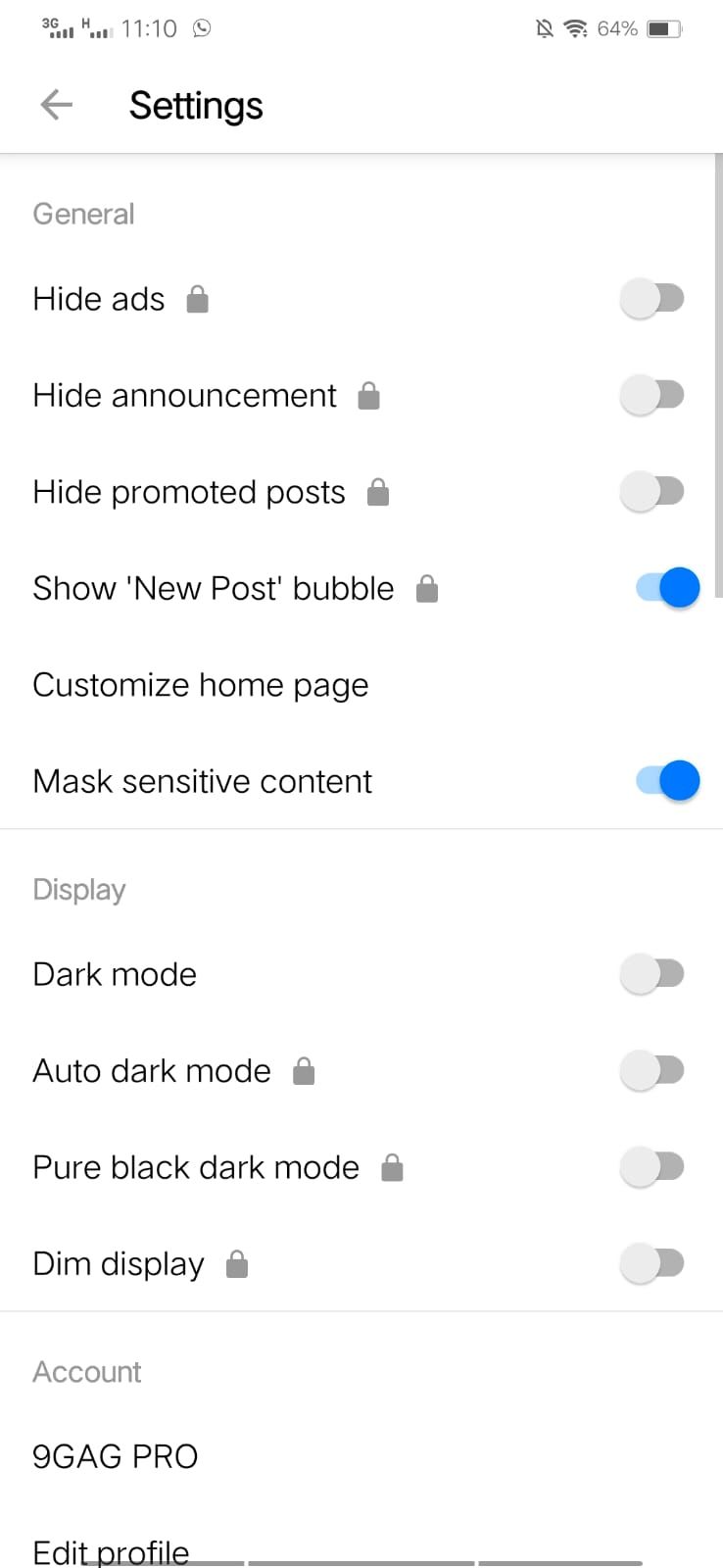A detailed image caption for the provided description could be:

---

The image shows a screenshot of a phone's settings menu with various toggle switches and icons. At the top of the screen, the status bar displays multiple icons including the time, a WhatsApp icon, a muted bell icon, a Wi-Fi icon, the battery percentage (64%), and a battery icon indicating the current charge level. Below the status bar, the title "Settings" is displayed alongside a back arrow and a dividing gray line.

The main section of the menu is headed by "General." The list of toggles under "General" is as follows:
- "Hide Ads" (untoggled, gray)
- "Hide Announcement" (untoggled, gray)
- "Hide Promote Posts" (untoggled, gray)
- "Show New Post Bubble" (toggled, blue)
- "Customize Home Page" (no toggle available)
- "Mask Sensitive Content" (toggled, blue)

A gray line separates the next section, which has the title "Display." The list of toggles under "Display" includes:
- "Dark Mode" (untoggled, gray)
- "Auto Dark Mode" (untoggled, gray)
- "Pure Black Dark Mode" (untoggled, gray)
- "Dim Display" (untoggled, gray)

Another gray separator bar follows, with gray text below it displaying "Account," "9GAG Pro," and "Edit Profile."

All text is black on a white background, making the interface clean and easy to read.